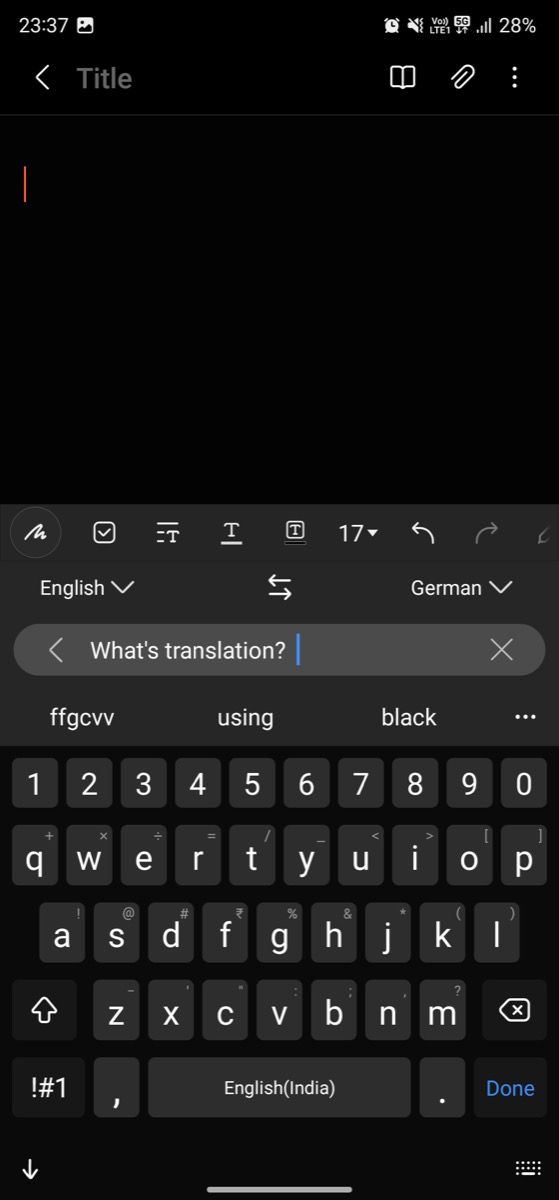In this richly detailed screenshot, we capture the user interface of a mobile device at exactly 11:37 AM. The upper left corner displays the current time, accentuating the device's settings. Adjacent to the time is the gallery icon, suggesting easy access to the user's photos.

On the upper right side, several status icons are present: an active alarm icon, indicating an alarm is set; icons signaling that the phone is on vibrate and mute; a VoLTE (Voice over LTE) icon; and a 5G signal strength indicator, showing a robust 4 out of 5 bars. Additionally, the battery charge indicator reveals a remaining battery life of 28%.

Dominating the central portion of the screen is a notepad application, presumably where the user jots down quick notes or important information. Highlighted here is the device's on-screen keyboard, featuring a text input area with the following content: "What's translation? Thanks for watching, and leave your comments here." This message hints at a possible query or engagement prompt, inviting feedback or responses from those viewing the content.